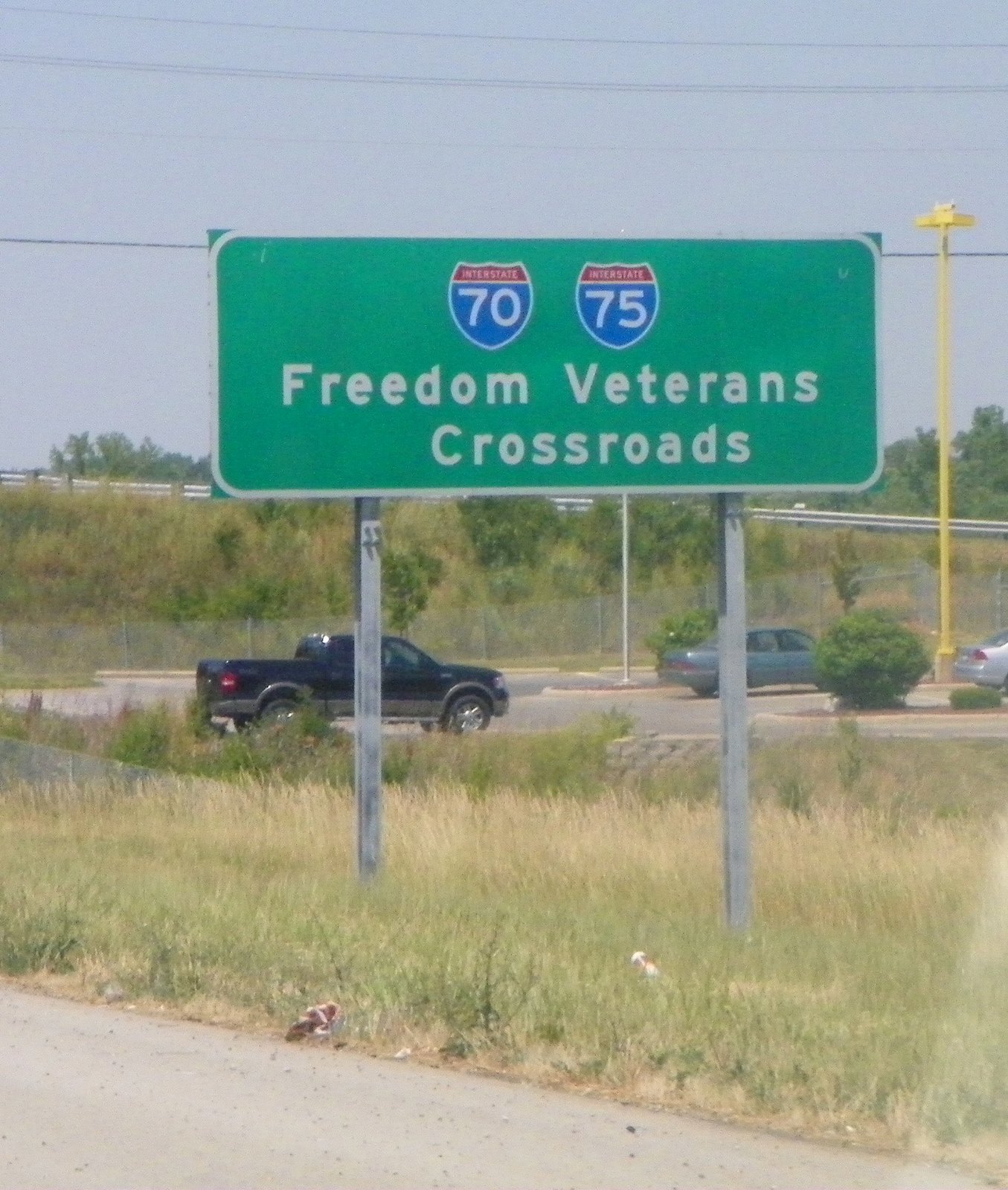The image depicts a bright daytime scene looking over an embankment covered with dry grass towards a main road or highway. Prominently in the foreground is a green street sign. This sign indicates "Freedom Veterans Crossroads" and displays the blue and red shield logos for Interstate 70 and Interstate 75. Below the sign, a stone wall and a metal railing are visible, separating the field from the highway. Beyond the embankment, the gray asphalt road hosts several vehicles, including a black truck, a blue sedan, and a white car. Nearby, a bright yellow light pole stands tall, with numerous power lines and telephone poles stretching into the distance. The scene is framed by a clear, light blue sky, highlighting the expansive and open nature of this roadway setting.